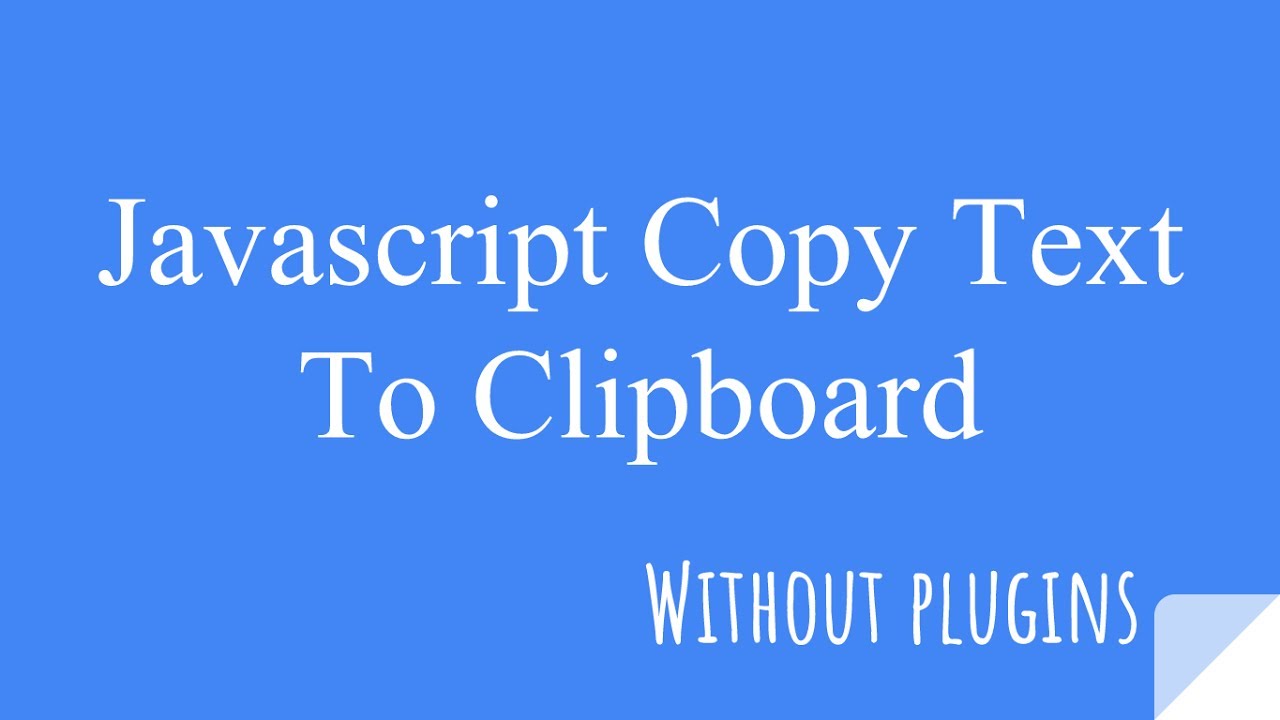This image features a clean, illustrative design set against a solid light blue background. The background square is predominantly blue with a light white section resembling folded dog-ear paper positioned at the bottom right corner, adding a subtle 3D effect. Centered within the blue, the text prominently displays the phrase "JavaScript Copy Text to Clipboard" with each word beginning with a capital letter. The font is modern and easily legible. Towards the lower right-hand corner, a bold message in a distinct font reads "WITHOUT PLUGINS," completely in uppercase, standing out clearly against the blue background.